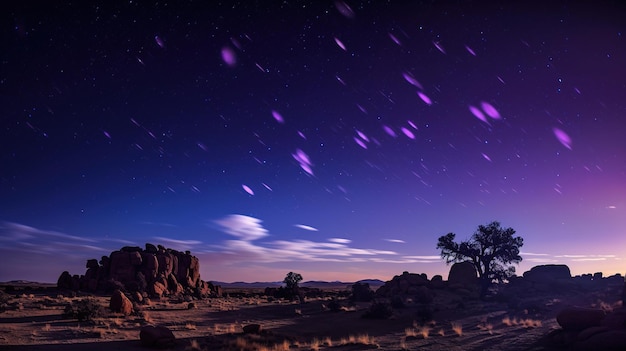The landscape photograph captures a stark desert scene under a mesmerizing twilight sky. Dominating the top half of the image, the sky transitions from a lighter orange near the horizon, filled with scattered white clouds, to deep hues of purple and dark blue, culminating in almost black near the top left corner. This celestial view is dotted with white specks representing stars, some appearing elongated as if captured in a time-lapse, and blurry purple dots that resemble distant clouds. The barren, rocky terrain below is sparsely vegetated, hosting a few small clumps of yellow grass and isolated trees with sparse leaves. The desolate ground stretches from left to right, with a rocky plateau of orange-tanned stones prominently featured towards the bottom left corner. Amidst the flat dirt and scattered boulders, one particularly lone tree stands out, silhouetted against the otherwise dimly lit landscape, a silent testament to the serene isolation of this nighttime desert vista.